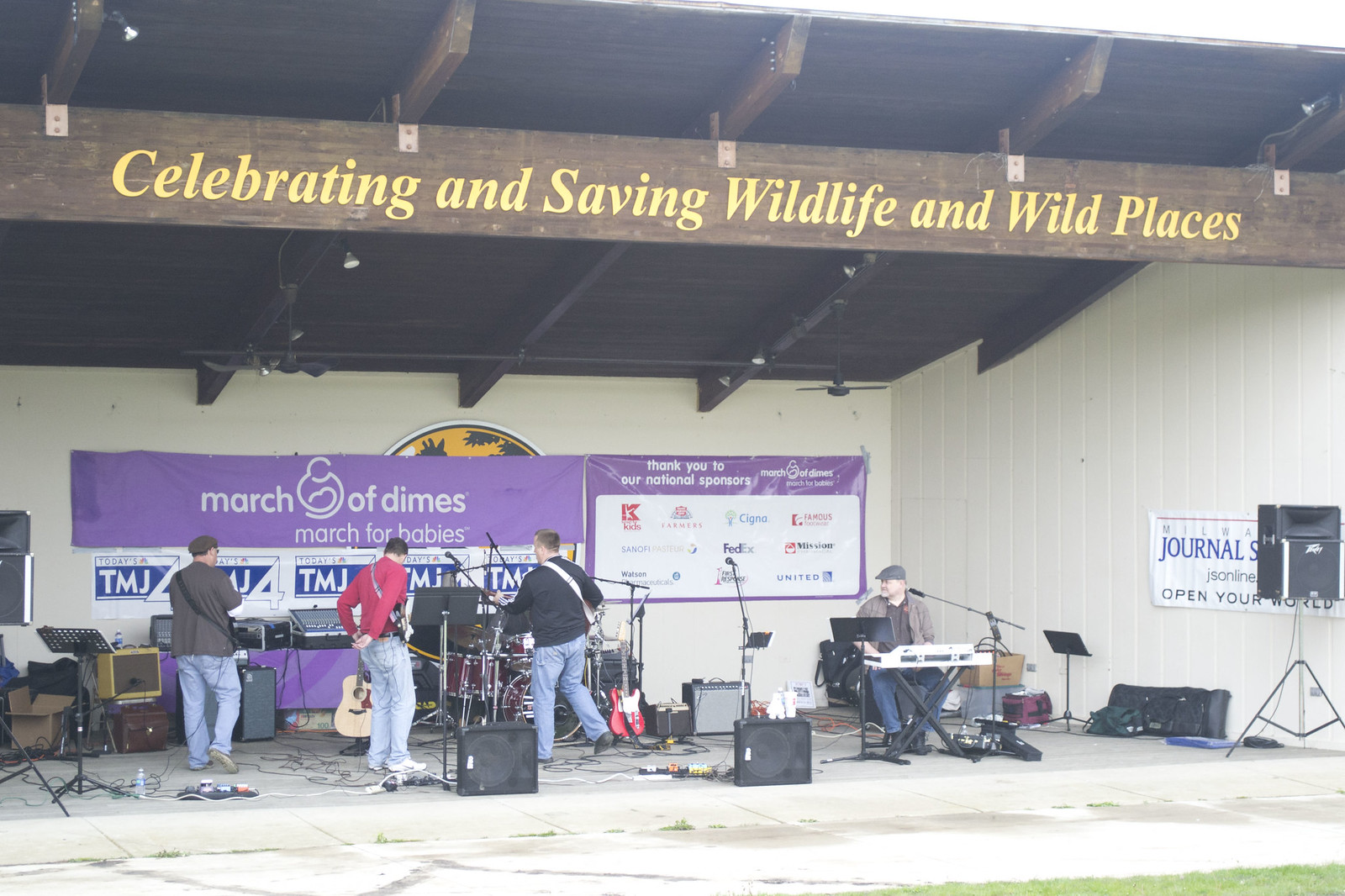In this vibrant daytime outdoor scene, a four-member band is captured amidst their performance, set against the backdrop of a stone-paved stage. Three men clutch guitars, while a fourth is seated at an electric keyboard. Amplifiers and speakers are positioned at their feet, suggesting a lively performance. Dominating the backdrop, a bandshell draped with a purple and white banner proudly displays the March of Dimes logo and the slogan "March for Babies," accompanied by acknowledgments to national sponsors. Above the performers, a prominent text beam reads "Celebrating and Saving Wildlife and Wild Places" in bold yellow letters. The image brims with color, featuring green, white, tan, blue, purple, yellow, gray, and brown hues, and encapsulates the spirited atmosphere of a charity event dedicated to supporting wildlife and children's health initiatives.